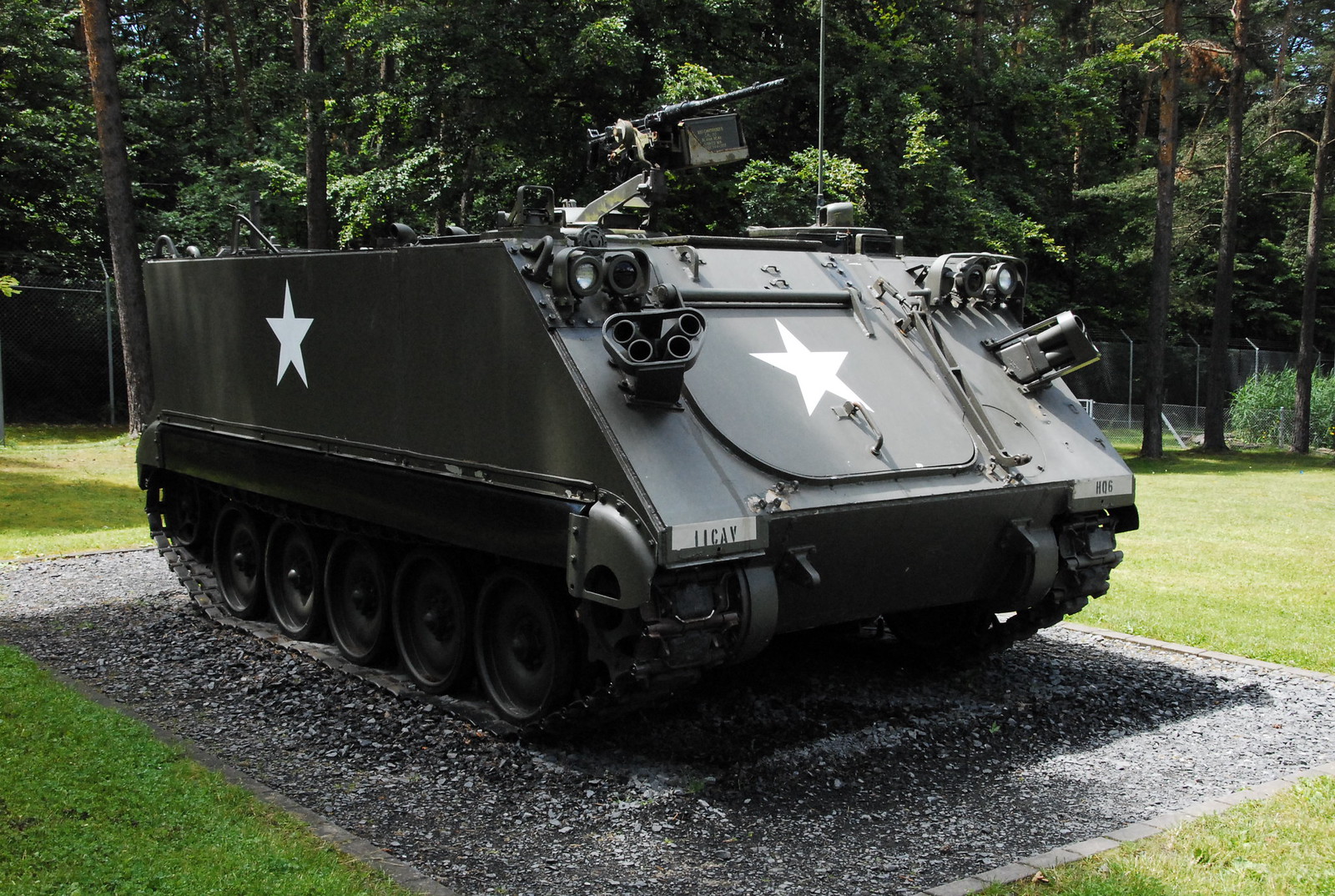This is a detailed photograph of a small, old-fashioned armored tank on display in a picturesque, forested setting. The tank, which appears to be from the 1950s, is predominantly black in color and features a prominent white star on both its front and left side. The vehicle is equipped with treads over its wheels and has various pieces of equipment attached, including a mounted gun on top and several protruding attachments such as headlights and possibly a bullhorn or sound amplifier.

The tank is positioned in the center of a rectangular garden filled with loose dark black and gray rocks and stones. Bright green grass surrounds this display area, providing a stark contrast to the dark hues of the tank and stones. In the background, large, tall trees with dark brown trunks and lush, bright green foliage dominate the scenery. Additional greenery, including a variety of vibrant shrubs, can be seen particularly on the right side of the image, contributing to the idyllic and verdant forest atmosphere.